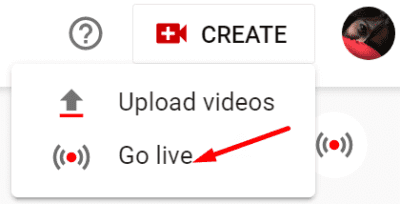The image features a clean white background with several distinct elements. On the left side, central to the composition, is a gray outlined circle containing a gray question mark. Adjacent to this is the faint outline of a rectangle. Inside this rectangle, in capital black letters, is the word "CREATE," positioned next to a small red square with a white plus sign, and a red triangle to its right.

Below this area, there is a profile picture presented in a circular frame. The details of the picture are unclear, featuring indeterminate red and dark brown colors that remain indistinguishable even when enlarged.

Overlaying this section is a white popup box containing the instructions "UPLOAD VIDEOS" written in gray, alongside a prominent thick arrow pointing upwards with a red line underneath. Below this, the option "GO LIVE" is presented in gray text. To the left of this option is an icon featuring two partial gray circles encasing a red dot, symbolizing live broadcasting.

Additionally, a large red arrow directs attention towards the "LIVE" section. In the backdrop of the popup box, the same circular broadcasting symbol—two gray half circles with a red dot in the middle—reappears, enhancing the thematic consistency of the image.